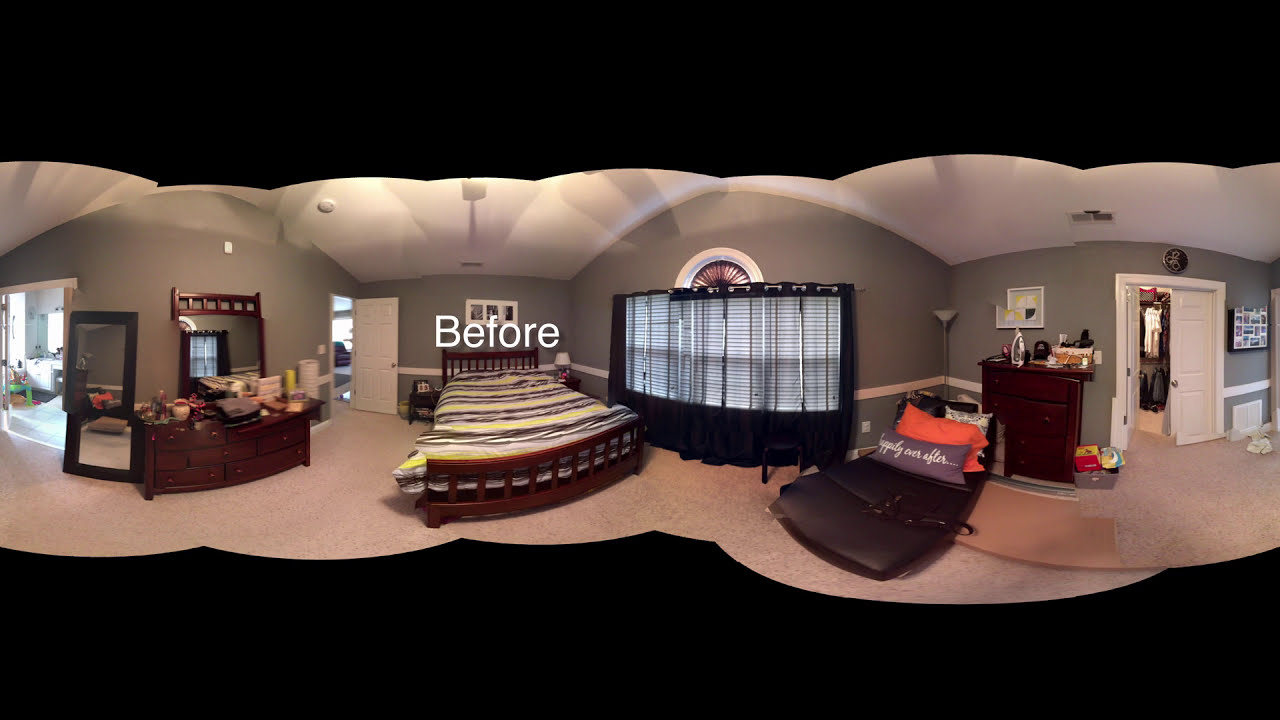In this image, we see a distorted, widescreen panorama of a bedroom that appears to have been stitched together from multiple photographs, resulting in a curvy, cloud-like shape bordered by black bars at the top and bottom. The bedroom has brown-beige/sage green colored walls and a white ceiling. The central focus is a bed with a brown frame and red and black striped sheets. The bed is positioned near a large window adorned with sheer black curtains. Above the bed, the word "before" is painted on the wall. To the left of the bed, there is a vanity with a mirror reflecting the window, and a brown dresser cluttered with items. In the left background, there are two large entrances leading to different rooms. On the right-hand side, the room features a leather mat or makeshift bed with multiple pillows, a small brown dresser piled with items, and white closet doors. Additional furnishings include tan or possibly hard flooring, another dresser, and various objects contributing to the detailed setting of this indoor scene, captured during the middle of the day. The colors in the room include black, tan, brown, gray, white, green, orange, and red.